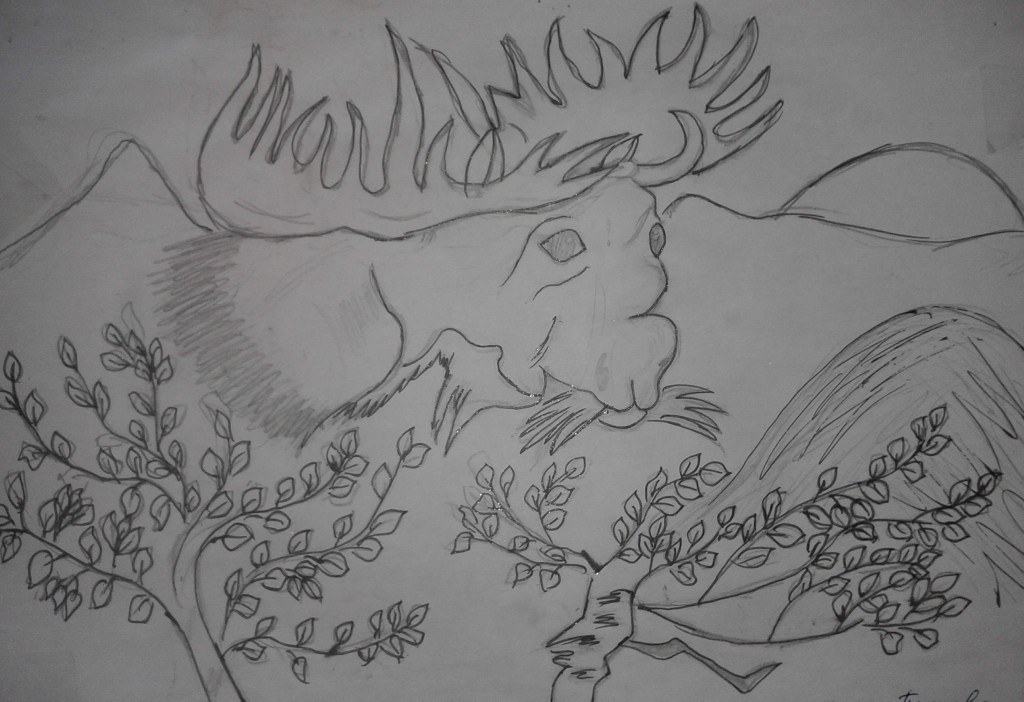This black and white pencil and pen drawing features a moose, centered slightly above the midpoint on a piece of white paper. The majestic animal is depicted with a detailed head and shoulders, its large antlers prominently framing its face. The moose is munching on grass or hay that hangs from its mouth. Its eyes are filled in with dark circles and faint pupils, giving it an expressive yet subtle look. 

In the background, a minimalist mountain ridge stretches across the scene, with a sun setting on the right side, casting a gentle glow over the landscape. In front of the moose, there's a small pile of hay, possibly the source of its meal. 

Two tree branches extend along the bottom edge of the paper. The branch on the left slants upward to the left and is adorned with flat, spade-shaped leaves. The branch on the right, likely from a birch tree, angles upward to the right, with simple leaf shapes and a distinctive trunk texture.

In the bottom right-hand corner, the faint top of an artist's signature can be seen, hinting at the creator’s identity and adding a personal touch to this intricately designed artwork.